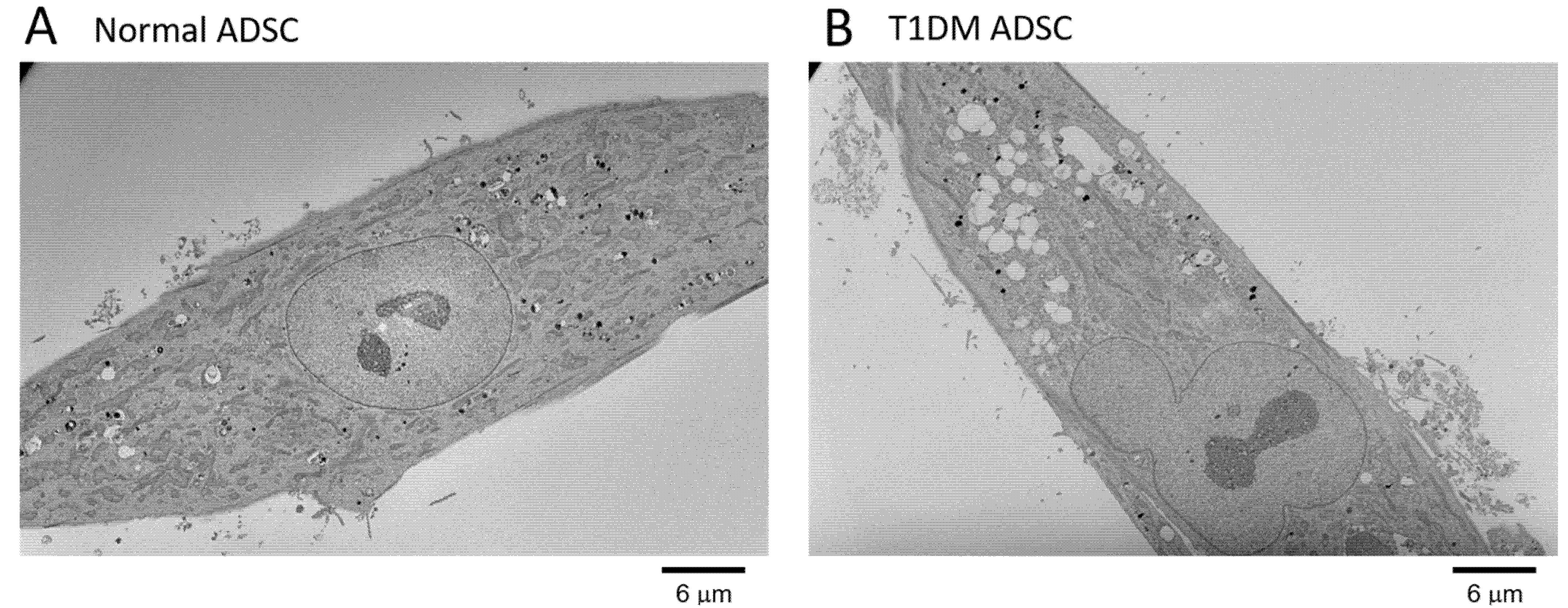The image depicts two grayscale graph pages labeled "A" and "B," each showcasing elongated, diagonal blobs on what appear to be gauze-like backgrounds. Page "A" on the left is titled "Normal ADSC" and displays a blob extending from the lower left to the upper right, while page "B" on the right is labeled "T1DM ADSC" and shows a blob stretching from the upper left to the lower right. Both pages feature a notation of "6 μm" at the bottom right corner, likely indicating a measurement scale of six micrometers. The background consists of intricately drawn horizontal and vertical lines, akin to standard graph paper. The blobs are distinguished by a slightly darker shade compared to the lighter gauze-like material. The image seems to originate from scientific research, potentially involving pathology or medical samples.